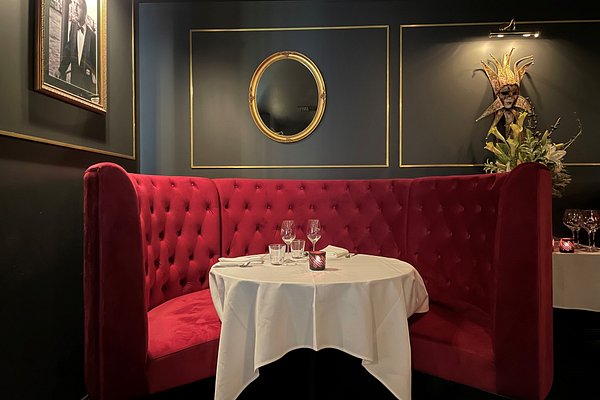The photograph captures an opulent corner booth in a luxurious restaurant. The rich brassy brown walls with dark brown accents provide an elegant backdrop. The booth features a curved, red velvet upholstered seat surrounding a round table draped with a pristine white tablecloth reaching down to the floor. On the table, two empty wine glasses and two shot glasses are placed alongside a small lit candle in a red holder. Two place settings showcase neatly arranged silverware atop napkins. Above the booth, a gold-framed portal-style mirror is highlighted within a square gold molding on the wall. To the right, another framed square molding features a light illuminating an aboriginal statue with lilies in front. Adjacent to the booth, on the left at waist height, hangs a brown-framed photograph of a man in a black tuxedo jacket and bow tie walking past some posts. The opulent atmosphere is further accentuated by the visible table beyond the booth, offering additional seating privacy for other diners.